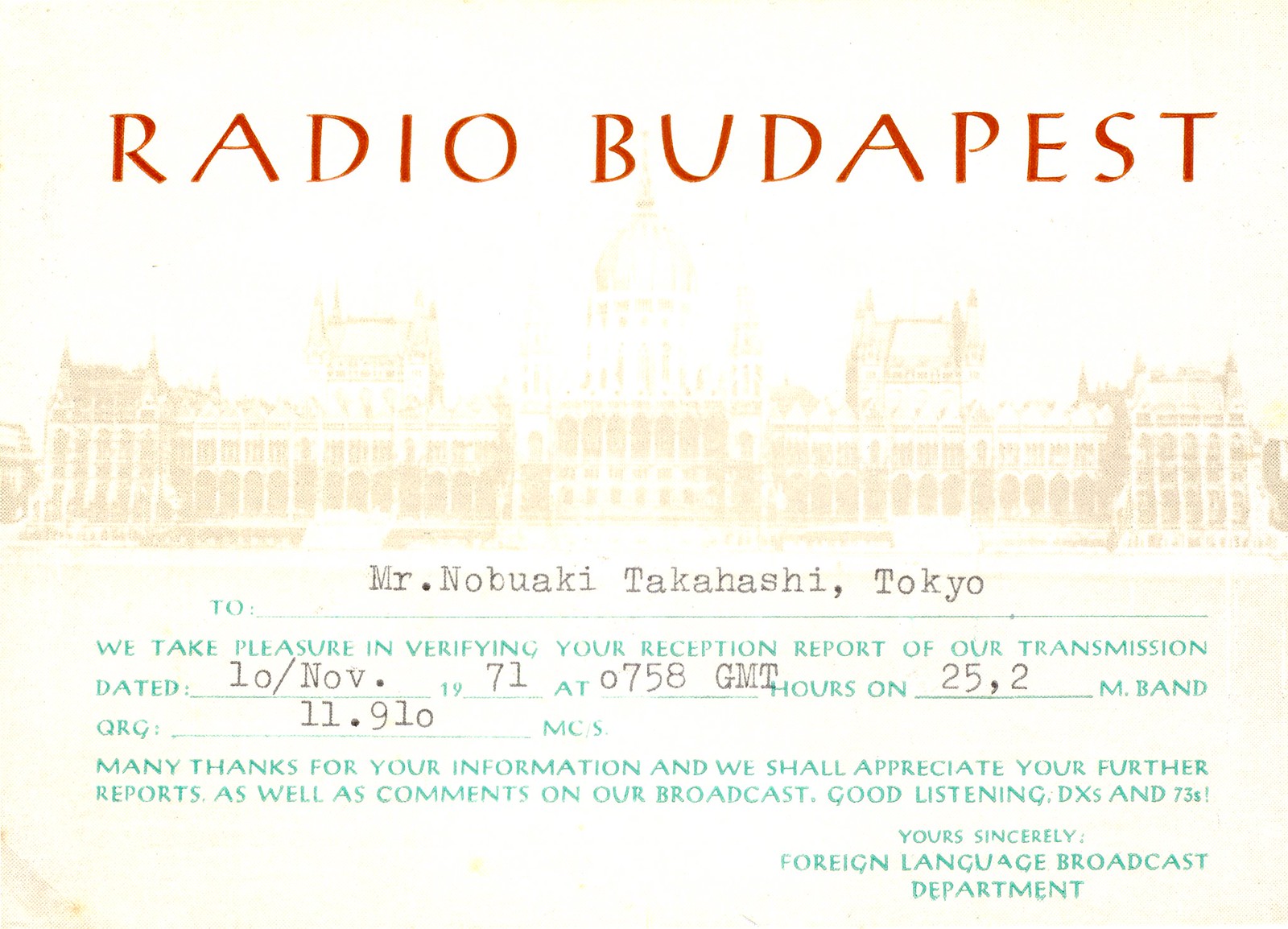The poster titled "Radio Budapest" features bold red capital letters across the top on a light yellowish background. Below the title, there is a faded image of a large, ornate building characterized by its broad structure, lined with columns, and a central tower capped with a golden dome. At the uppermost section, typewritten text in black addresses "Mr. Nobuaki Takahashi, Tokyo." Beneath the illustration, a green typewritten message reads:

"We take pleasure in verifying your reception report of our transmission dated 10 November 1971 at 0758 GMT hours, 25, 2M band origin 11.910 MCS. Many thanks for your information, and we shall appreciate your further reports as well as comments on our broadcast. Good listening, DXs and 73s. Yours sincerely, Foreign Language Broadcast Department."